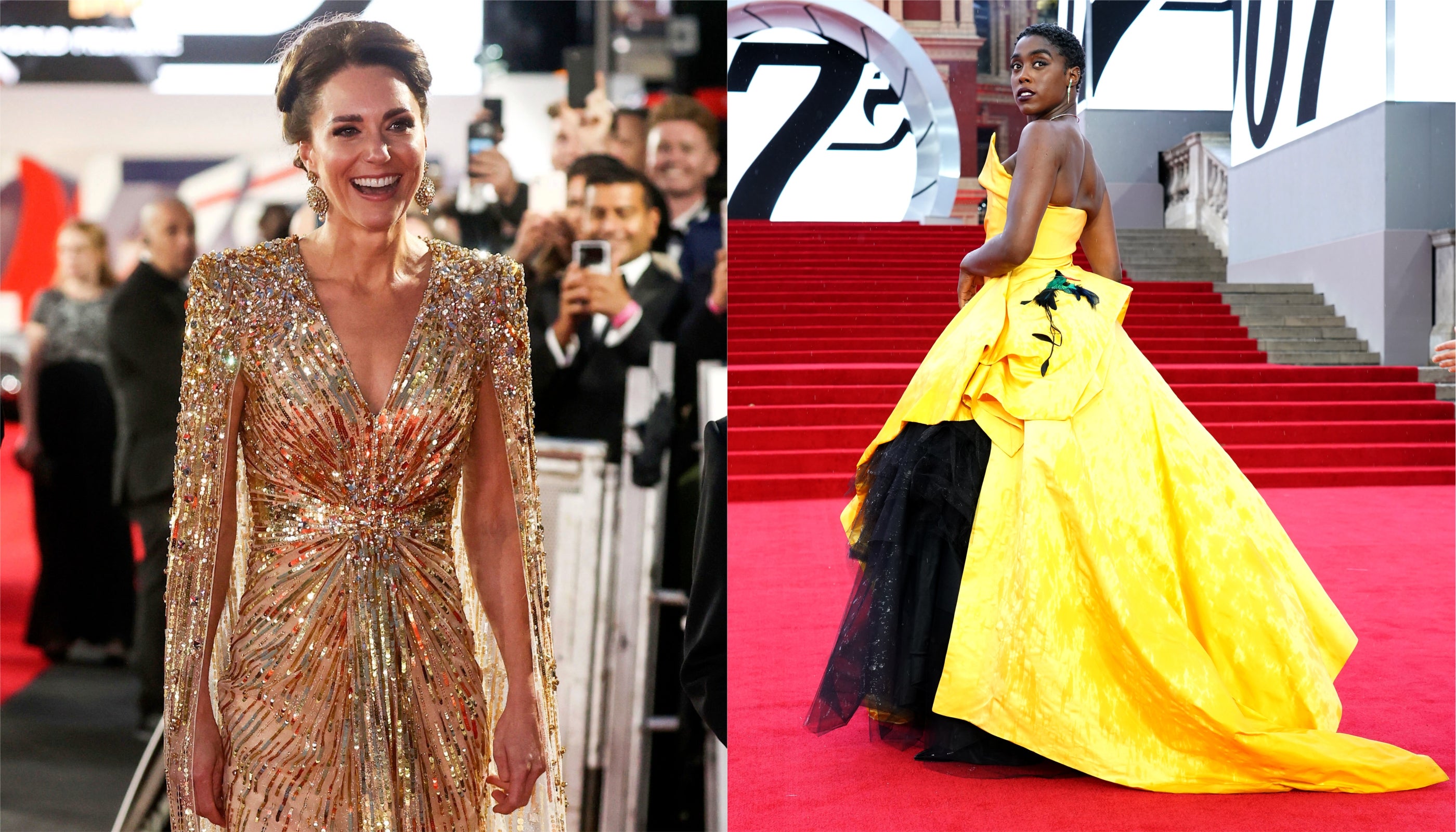This image features a composite of two side-by-side photographs, both capturing moments on red carpets at a luxurious event. On the left side, Princess Kate of the British royal family is beaming with joy, dressed in an elegant gold gown with cape-like long sleeves, a deep V-neck, and her hair pulled back. She accessorizes with gold earrings, and her joyous expression suggests she is engaging with the crowd behind her, who are eagerly snapping pictures on their cell phones. On the right side, actress Jodi Turner-Smith is poised at the base of a staircase, donning a stunning strapless yellow dress adorned with black tulle under the skirt. She stands confidently, glancing back towards the camera with a serene expression. The background and setting allude to an extravagant event, perhaps a movie premiere or a gala, underscored by the presence of red carpets, photographers, and the text "007" on the walls nearby. The overall scene is rich in vibrant colors including white, gold, yellow, black, and red, encapsulating the glamour and excitement of the moment.